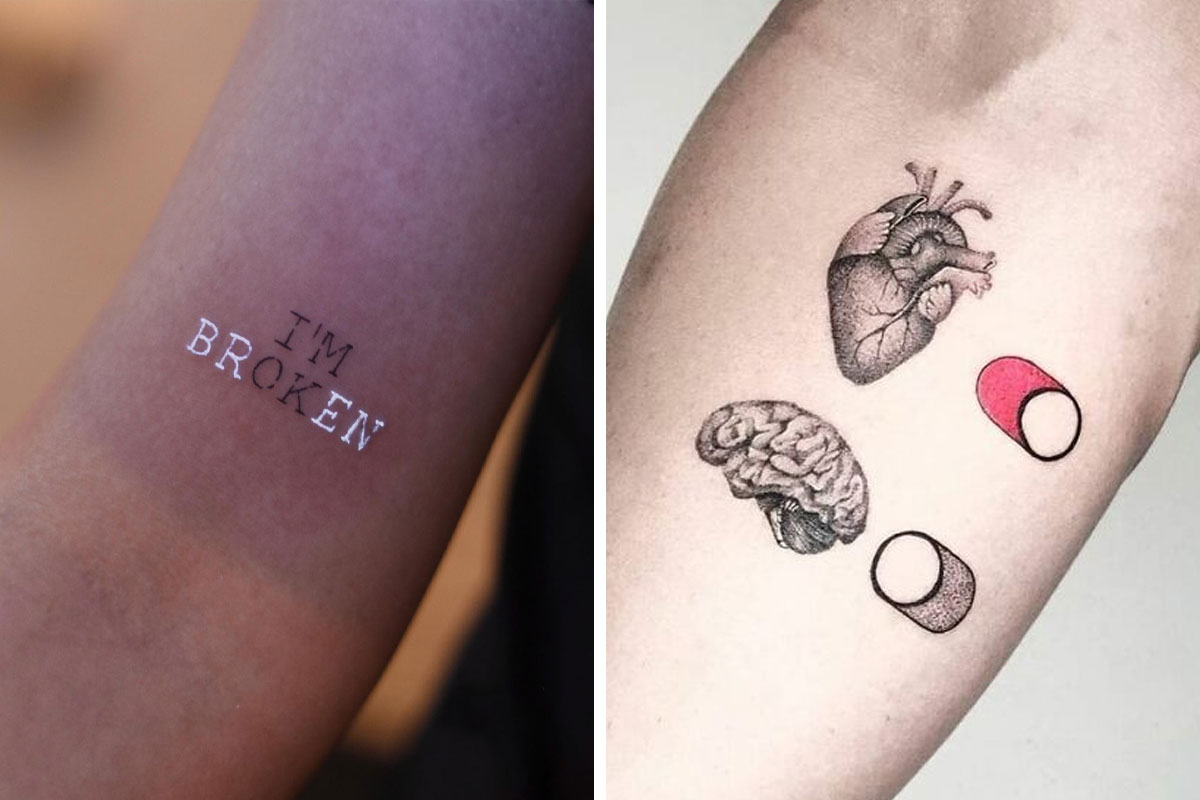This image showcases two distinct tattoos, one on each of two different forearms set against contrasting backgrounds. The left tattoo is a clever text-based design that reads "I'm broken" with certain letters—B, R, E, N—inked in white. This visual trick reveals "I'm okay" in black ink within the phrase. The background is a blurry brown and the arm's skin tone is light pink. The right tattoo is an anatomically detailed black-and-white rendering featuring a heart and a brain accompanied by toggle switches, suggesting that the heart is "on" (indicated by a red setting) while the brain is "off." This arm contrasts sharply with a whitish-gray background and includes cartoonish elements resembling pill halves, one red and white, the other gray and white. The juxtaposition of these tattoos captures contrasting themes of emotional complexity and the interplay between heart and mind.